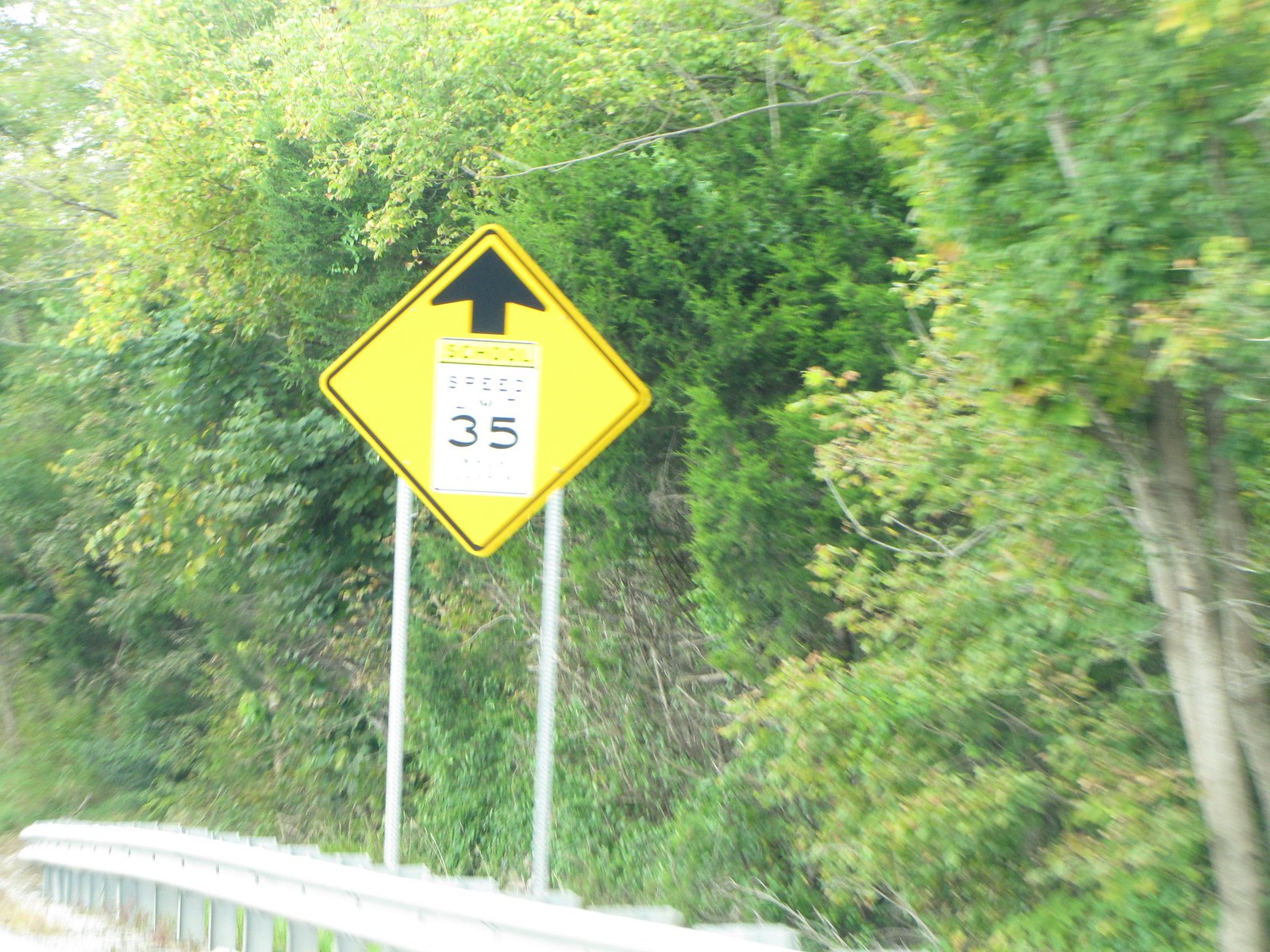The image captures the side of a road on a sunny day, featuring a stretch of metal guardrail running parallel to the street. Prominently positioned behind the guardrail is a vivid yellow diamond-shaped sign, held aloft by two slender white poles. This sign, bordered in black, displays a black arrow pointing upwards, and beneath the arrow, the word "school" is followed by a white box containing the number 35 in black. Flanking and extending beyond the sign is a dense, impenetrable thicket of green and yellow foliage, composed of trees with gray trunks and some leafless branches. The foliage is so thick that it obscures any view of the sky, emphasizing the lush, overgrown nature of the setting. The overall composition suggests that the photo was likely taken from a car window, capturing the natural and man-made elements of this roadside scene.